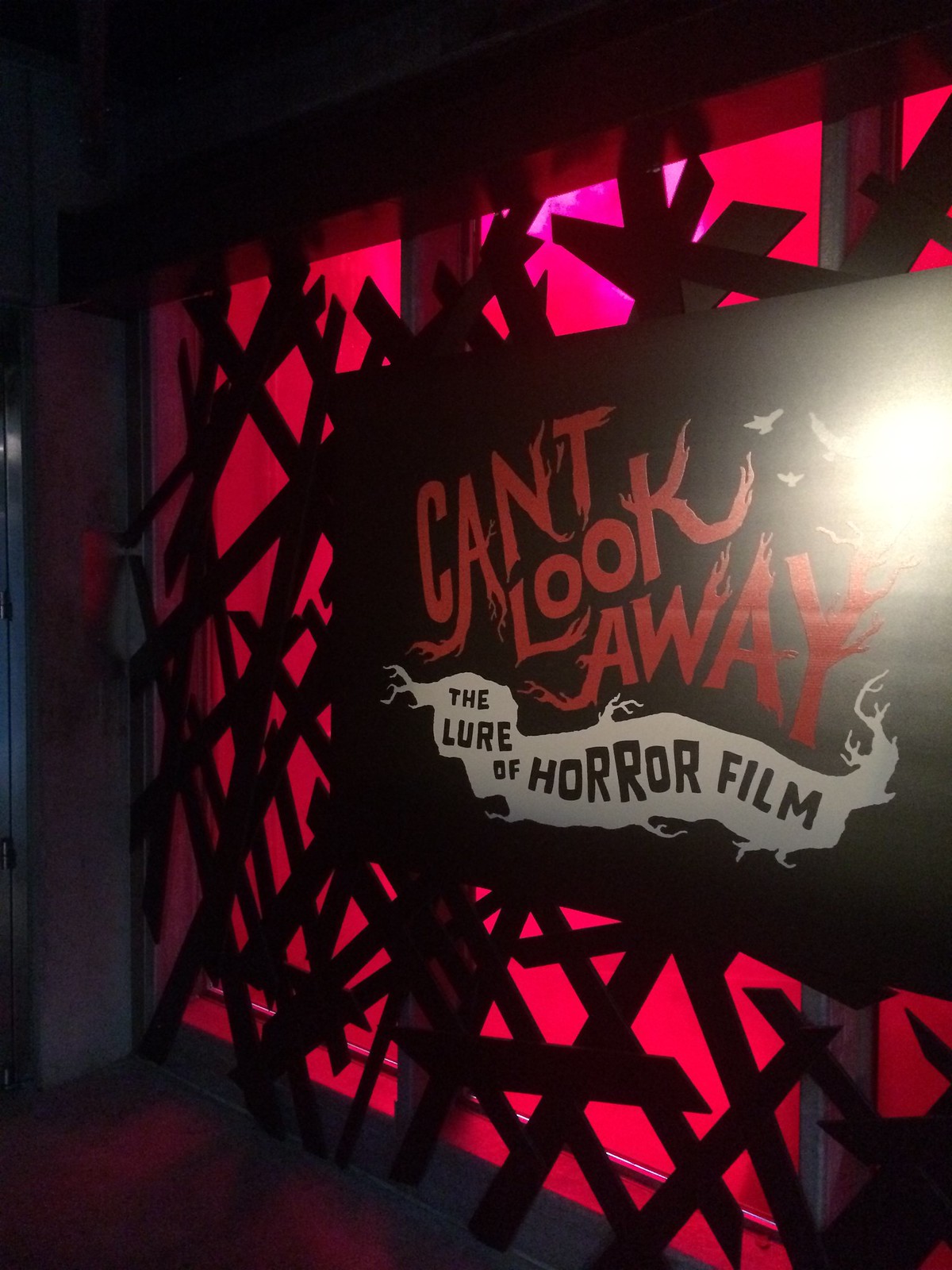The image depicts an eerie, indoor scene resembling a haunted house or horror film setting. The background is dominated by crisscrossing black bars, behind which emanates a glowing red and pink light, adding to the ominous atmosphere. At the center, a large black sign prominently features jagged, blood vessel-like red lettering stating "Can't Look Away." Below this, a white banner with black letters reads "The Lure of Horror Film." Above the text, white birds can be seen, and a bright yellow light illuminates the upper right corner, further emphasizing the spooky theme. The interplay of black, red, and ominous glowing lights creates a chilling and foreboding environment.